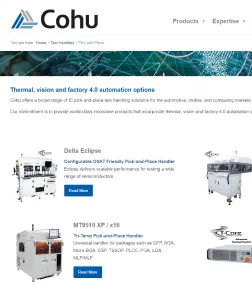The image depicts a webpage from a site called Kohu. Dominating the top left corner is a clever logo, intricately designed around a triangle that subtly incorporates the letters "C" and "H." To the right of the logo, the name "Kohu" is prominently displayed. On the right side of the page, a grey menu features a dropdown for "Products" and another for "Expertise," along with additional headings in a smaller, harder-to-read font.

Beneath this menu, a small banner with a generic green background serves to divide the screen. Below the banner, a vibrant blue heading reads "Thermal Visions and Factory 4.0 Automation Options." Accompanying this heading is grey text providing further details. 

The image showcases several pieces of industrial equipment. One section, labeled "Delta Eclipse," sits next to a second piece of machinery identified as the "M29510XP." Both items are accompanied by blue buttons, likely labeled "Read More," offering additional information upon clicking.

To the right of these pieces of equipment, two more machines are similarly showcased, completing the detailed overview of the webpage.